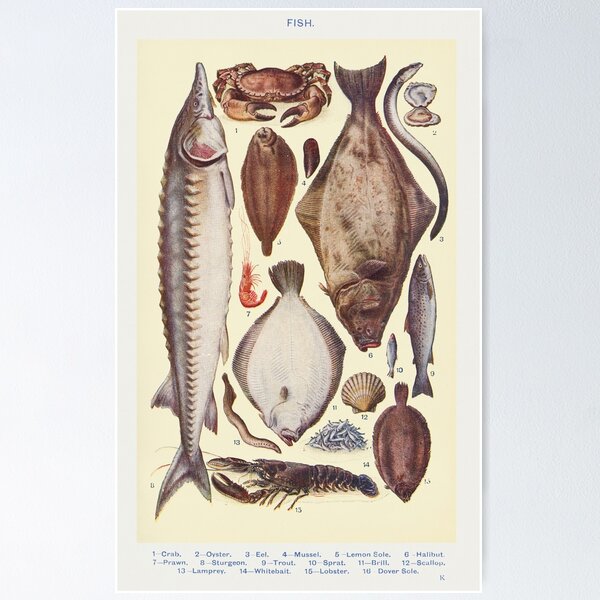The image depicts a lithographic print of various fish and nautical creatures set against a yellowish background with a white border. The detailed drawings, typical of late 18th to early 19th-century style, include creatures like a long oblong fish with scales and a dorsal fin on the left, a crab, a flounder, a curled eel, additional flat fish, a shrimp, and a lobster at the bottom facing left. Each illustration is numbered and labeled in small black text along the bottom white frame, corresponding to names such as crab (1), oyster (2), eel (3), mussel (4), lemon sole (5), halibut (6), prawn (7), sturgeon (8), trout (9), sprat (10), brill (11), scallop (12), lamprey (13), whitebait (14), lobster (15), and dover sole (16). While the background of the space where the poster is displayed is a solid light gray, the print itself is captioned "FISH" in bold black letters at the top, with the various sea creatures meticulously arranged in a lithograph style of gray and white sketches.